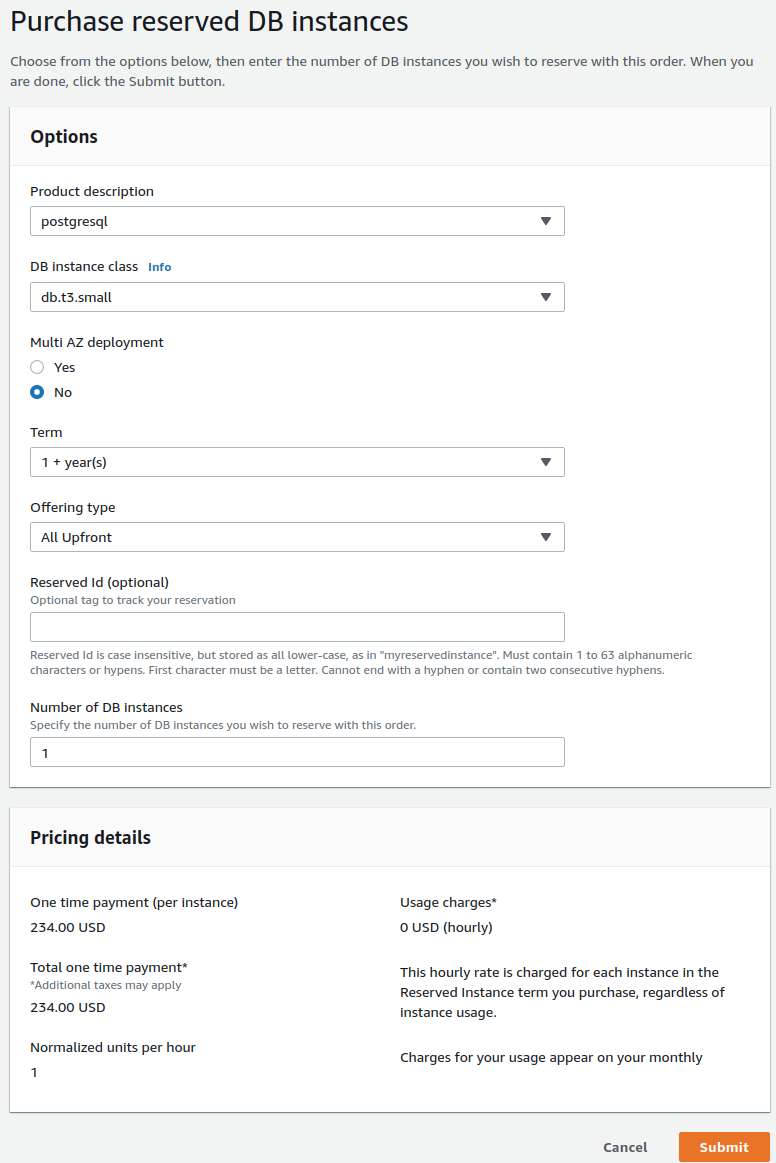The image displays a user interface for purchasing Reserved DB Instances. At the top, "Purchase Reserved DB Instances" is prominently shown in black text. Below this heading, instructions are provided: "Choose from the options below, then enter the number of DB instances you wish to reserve with the order. When you are done, click the Submit button."

Following this, the section titled "Options" includes several sub-sections. Under "Options," you find "Product Description" and "DB Instance." Underneath these, in very small text, "Multi-AZ Deployment" is displayed with a blue circle highlighting "No" as the selected option.

Further down, the "Terms" field allows for a selection of "three plus years." The "Offering Type" is set to "all up front." The interface also includes a section for a "Reserved ID (Optional)," followed by a blank area where text can be entered.

Towards the bottom, a section labeled "Pricing Details" contains several pieces of key information. It lists a "One-Time Payment" of "254 USD," repeated again under "Total One-Time Payment." Lastly, "Normalized Units Per Hour" shows the number "1."